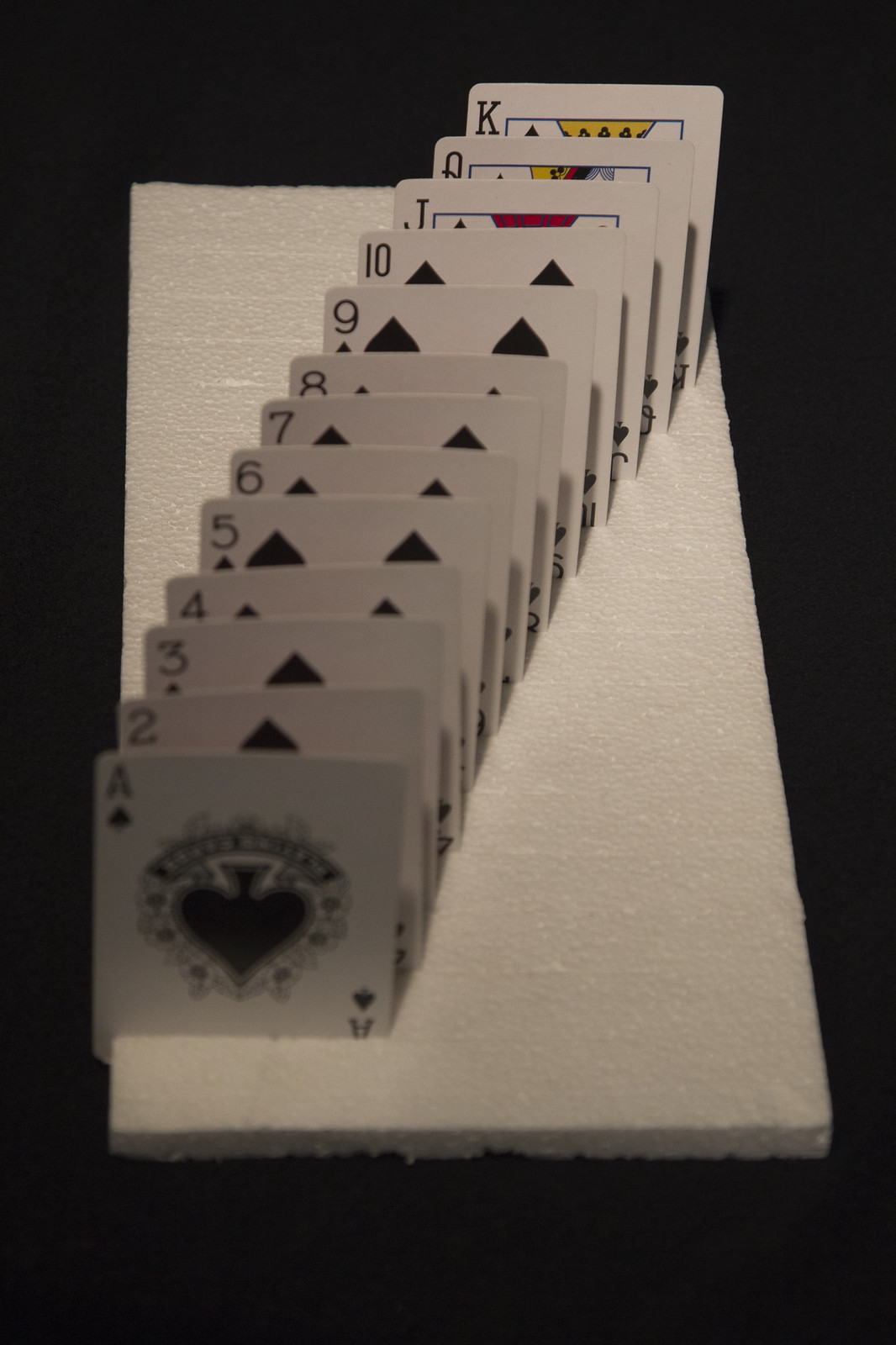The photograph features a striking composition set against a pitch-black background, casting full attention on the subject illuminated from both the top and front. At the center is a large, perfectly cut square of white Styrofoam. This Styrofoam square has meticulously crafted, diagonal slots running from the lower left corner to the upper right. Occupying these slots are a complete sequence of playing cards from the spade suit, each card placed upright. Beginning with the ace of spades nearest to the viewer, the cards progress in numerical order up to the king of spades. The pristine white of the Styrofoam contrasts sharply with the vibrant designs on the cards, making each card—ranging from the ace through the numerical cards and culminating in the face cards of jack, queen, and king—clearly visible and distinct. This thoughtful arrangement and dramatic lighting effectively highlight both the texture of the Styrofoam and the intricate details of the playing cards.